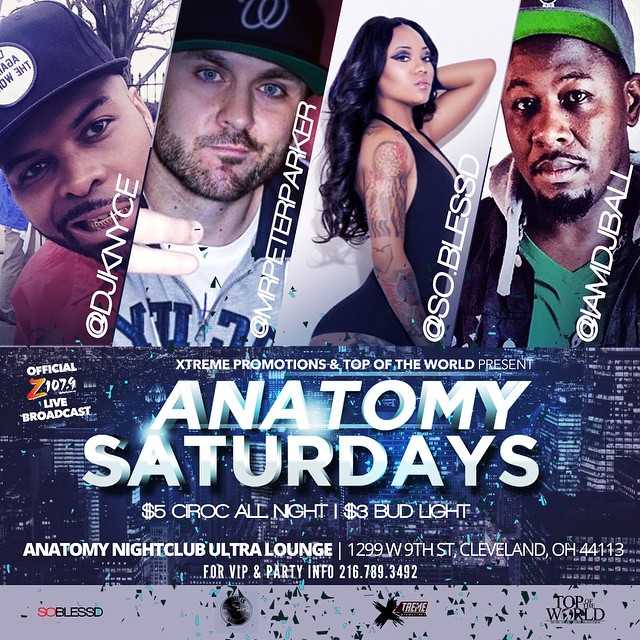This promotional poster for Anatomy Nightclub Ultra Lounge advertises 'Anatomy Saturdays,' featuring a striking design with 3D-lit white text. The top portion of the poster is divided into four diagonal sections, each highlighting a different individual:

1. The far-left section showcases @DJ KNYCE, who has a thin mustache and beard and wears a black cap.
2. Next to him, @MrPeterParker is depicted, also with a thin mustache and beard, blue eyes, and a black cap with a white logo.
3. The third section features @so.blessed, a woman in a tight black dress with visible tattoos on her right arm. She sports heavy blue eyeshadow and has long black curly hair.
4. Finally, @IMDJBALL appears in the far-right section, wearing a green shirt and a ball cap, with thin facial hair.

Beneath these pictures, the poster highlights the event details: 'Anatomy Saturdays' are presented by Extreme Promotions and Top of the World, offering $5 Ciroc all night and $3 Bud Light. The venue is Anatomy Nightclub Ultra Lounge, located at 1299 West 9th Street, Cleveland, Ohio 44113. For VIP and party info, interested parties can contact 216.789.3492. Additional sponsor logos are displayed at the poster's bottom.